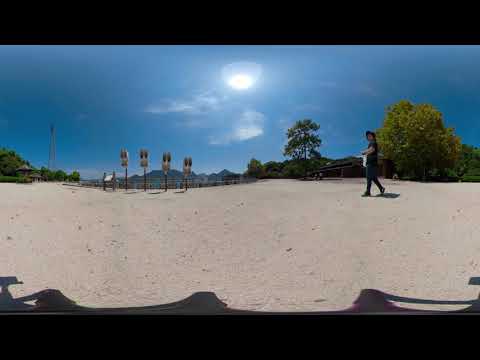In this computer-generated image, a woman dressed in black pants and a short-sleeved black shirt walks on a sandy landscape. Positioned towards the right side of the image, she moves from right to left. The scene is framed by thick black borders at the top and bottom. The sandy expanse occupies the lower portion, while a midsection of the image features a backdrop of trees and a fence. To the left center, there are four black poles with rectangular tops, slightly blurred. Near these structures, lower wooden supports are visible. In the distant background, a range of mountains extends across the horizon. The sky, occupying the top part of the image, is a mix of blue with gray and white clouds, with the sun peeking through. The scene is awash in colors: black, tan, gray, green, blue, and white, suggesting a tranquil outdoor setting on a sunny day.